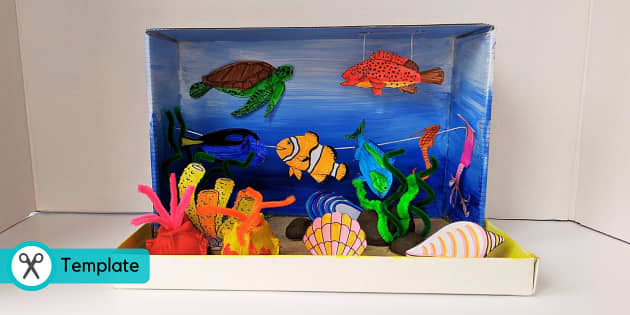This image showcases a detailed underwater scene diorama made from a shoe box. The diorama is arranged with the lid acting as the ocean floor, painted yellow and adorned with seashells and colorful coral made from pipe cleaners in pink and yellow hues, as well as an illustrated background of orange and yellow coral. The box is painted in gradients of blue, with darker shades at the bottom and lighter hues at the top, mimicking ocean depths. The sea life includes a vibrant green turtle with a brown shell, an orange and white clownfish, a red fish with black speckles and brown fins, and a blue fish with green markings around its eyes and sides. Additionally, there's a blue fish resembling Dory from Finding Nemo. The box is placed against a white background, with a transparent overlay at the bottom left showing scissors and the word "template."